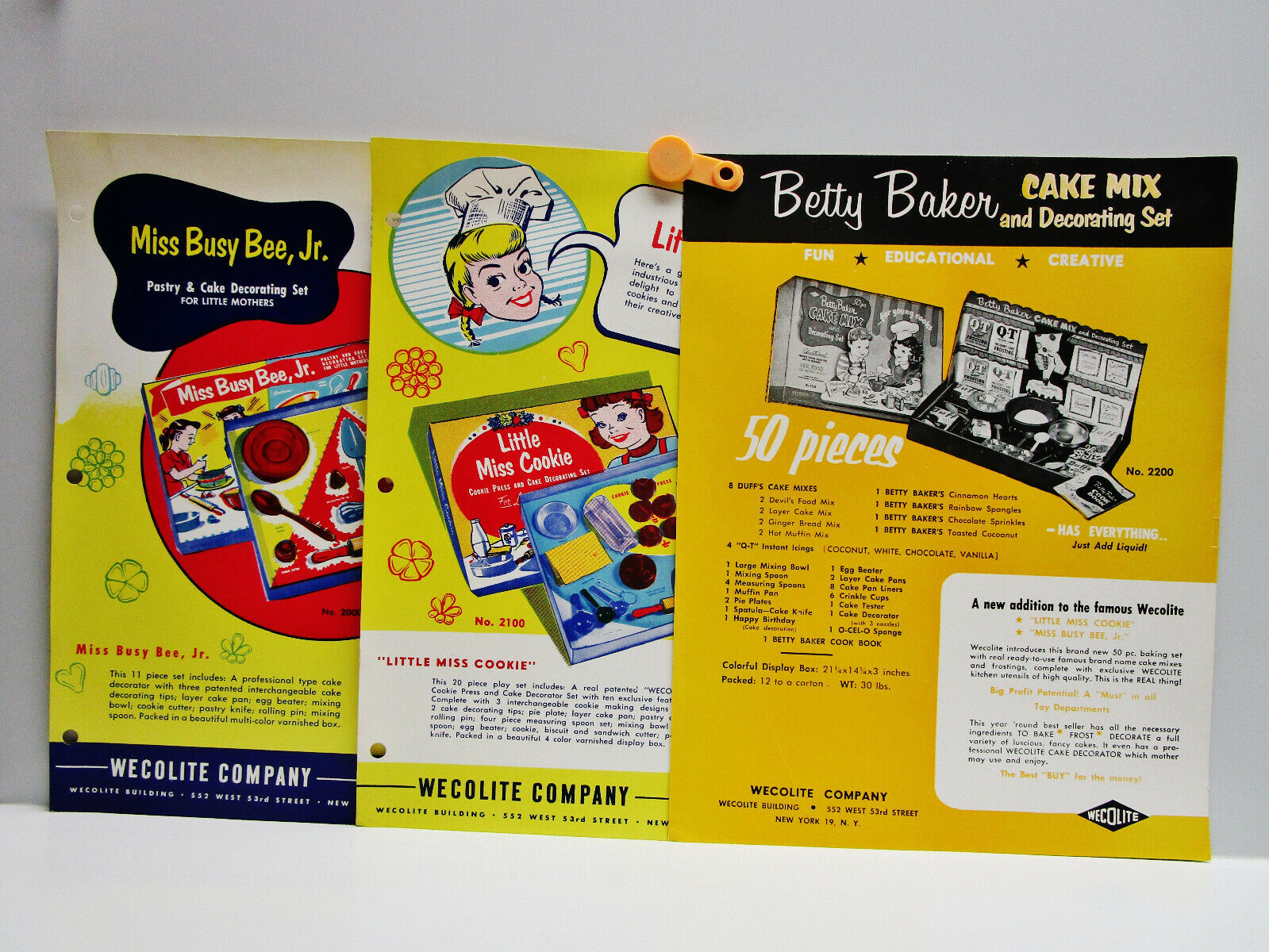This image showcases the back of several vintage magazine ads from the 1950s or 1960s. Dominating the scene is a vivid mustard-yellow advertisement for the "Betty Baker Cake Mix and Decorating Set," a comprehensive kit featuring 50 pieces, including real, ready-to-use cake mixes and frostings, along with exclusive Weekoblite kitchen utensils. The design is typical of the era, with intricate and somewhat cluttered layouts. The ad is split into sections, displaying a closed box and then an open one, revealing the various components. Adjacent to this, partially obscured, is an ad for "Little Miss Cookie," another child-oriented product by Weekoblite, featuring a young blonde girl in a chef’s hat alongside various baking tools. On the left, a portion of the "Miss Busy Bee Jr." advertisement is also visible, hinting at yet another playset from Weekoblite. Though each ad is partially covered, the overall imagery and color schemes reflect a nostalgic and highly detailed marketing style of the mid-20th century.